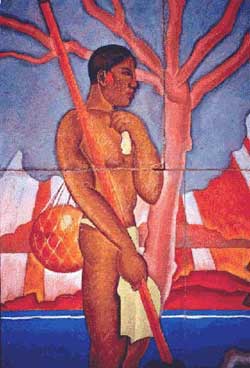The painting resembles an old postcard with a visible horizontal crease across the center. It vividly depicts a Native American man of brownish skin tone standing in front of a stark, leafless tree with a blue sky and distant hills in the background. The man, seen from his right profile, is almost bare except for a white loincloth. He has short, dark hair with a red marking near his ear, possibly an ear decoration. In his right hand, he holds a long wooden staff that leans across his right shoulder, balancing a net containing an orangish ball. His left arm is bent at the elbow, with his hand resting thoughtfully under his chin. The tree behind him is thin and barren, while the body of water at the bottom of the image, painted in dark blue hues, completes the serene yet solitary setting against a backdrop of flat-colored cliffs and a clear sky.